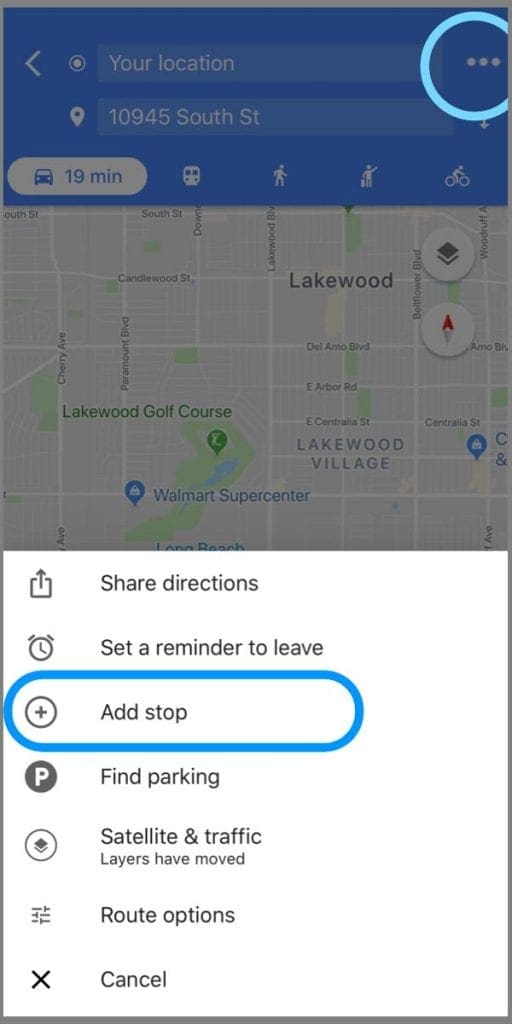The top of the image features a blue border and a box indicating the user's location, specified as "10945 South Street." To the right of this location box, there is a horizontal ellipsis encircled by a light blue oval. Below this, a Google Maps screenshot displays the area of Lakewood, highlighting notable landmarks such as the Lakewood Golf Course, Walmart Supercenter, and Lakewood Village. The bottom section of the image has a white background with a series of icons aligned to the left. Next to each icon, there is corresponding text listed vertically from top to bottom: "Shared direction," "Set a reminder to leave," "Add stop," "Find parking," "Satellite and traffic," "Layers have moved," "Route options," and "Cancel." The text "Add stop" is specifically circled with a light blue line.